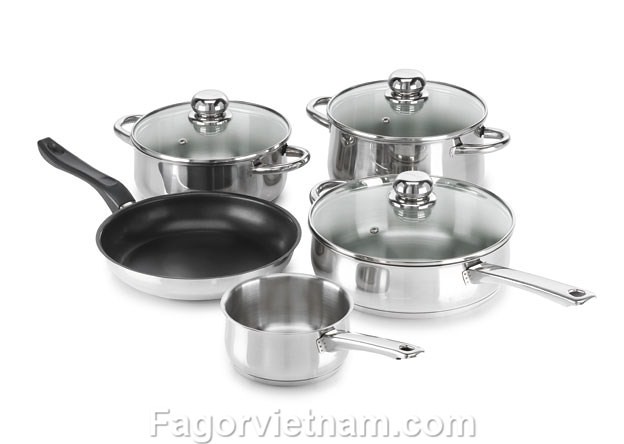This image showcases a promotional photograph of a five-piece set of pots and pans, prominently featuring a URL at the bottom, fagorvietnam.com, indicating that it is likely from an online store specializing in cookware. The arrangement includes a variety of stainless steel cooking implements against a clean, white background which enhances their shiny, silver finish. Starting from the back, there are two large pots with silver handles and clear glass lids topped with stainless steel knobs. At the front center, there is a small saucepan with a single silver handle facing to the right. On the left side of the arrangement, there is a black non-stick frying pan with an aluminum or steel exterior. On the right side, a larger high-sided pan with a long silver handle is also covered by a glass lid. All pieces appear new and are likely part of a digital catalog featuring high-quality kitchen appliances available for purchase from FagorVietnam.com.